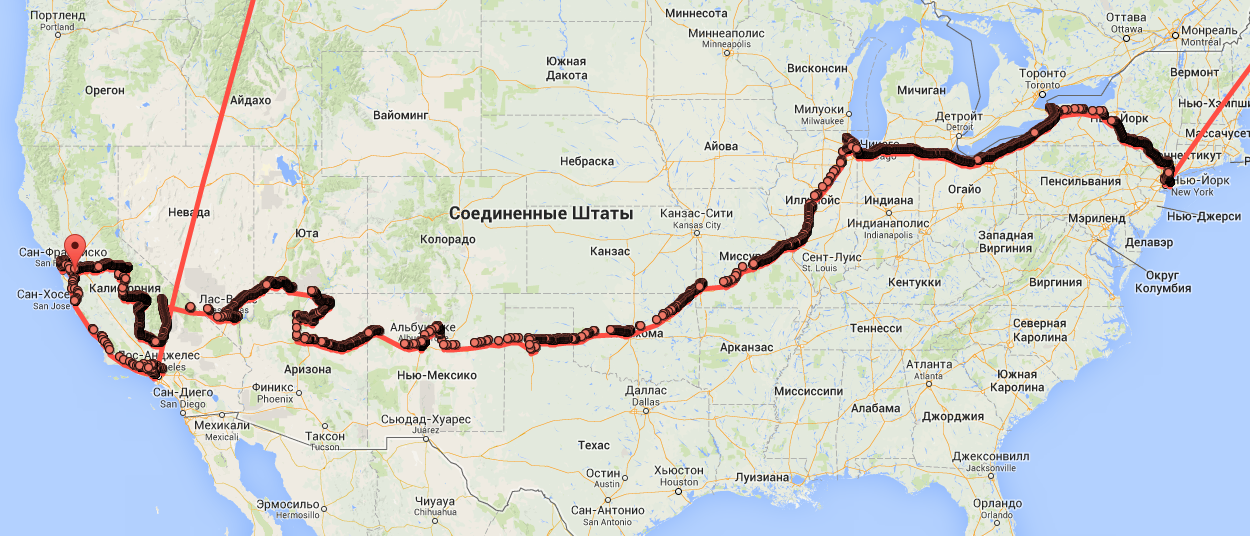This detailed image showcases a map of the United States of America, traversed by a prominent red path stretching from New York to California. Intriguingly, all the city and state names across the country are labeled in Russian, adding a layer of unusual and striking cultural juxtaposition to this visual representation. The path vividly cuts through the diverse geographical landscape, providing a stark contrast to the Cyrillic text that denotes familiar locations in an unfamiliar script.